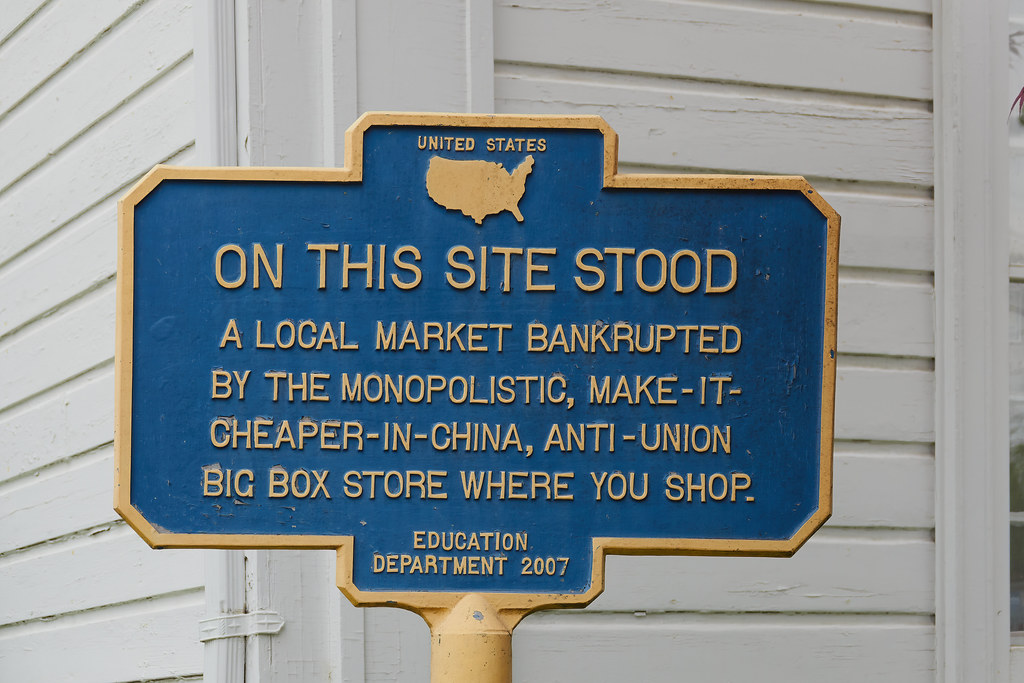The image depicts a metal historical marker sign with a blue backdrop and a yellow (or gold) border, resembling those often found at state parks or historical sites. The sign is positioned against the backdrop of a white wooden building, the corner of which is visible behind the marker. At the top center of the sign, in small text, it reads "United States," accompanied by a cutout map of the United States in yellow. The main text, prominently displayed in yellow, states: "On this site stood a local market, bankrupted by the monopolistic, make it cheaper in China, anti-union, big box store where you shop." At the bottom, in smaller yellow text, it reads, "Education Department, 2007." The message of the sign is notably aggressive and political, highlighting the adverse effects of monopolistic practices and the global supply chain.